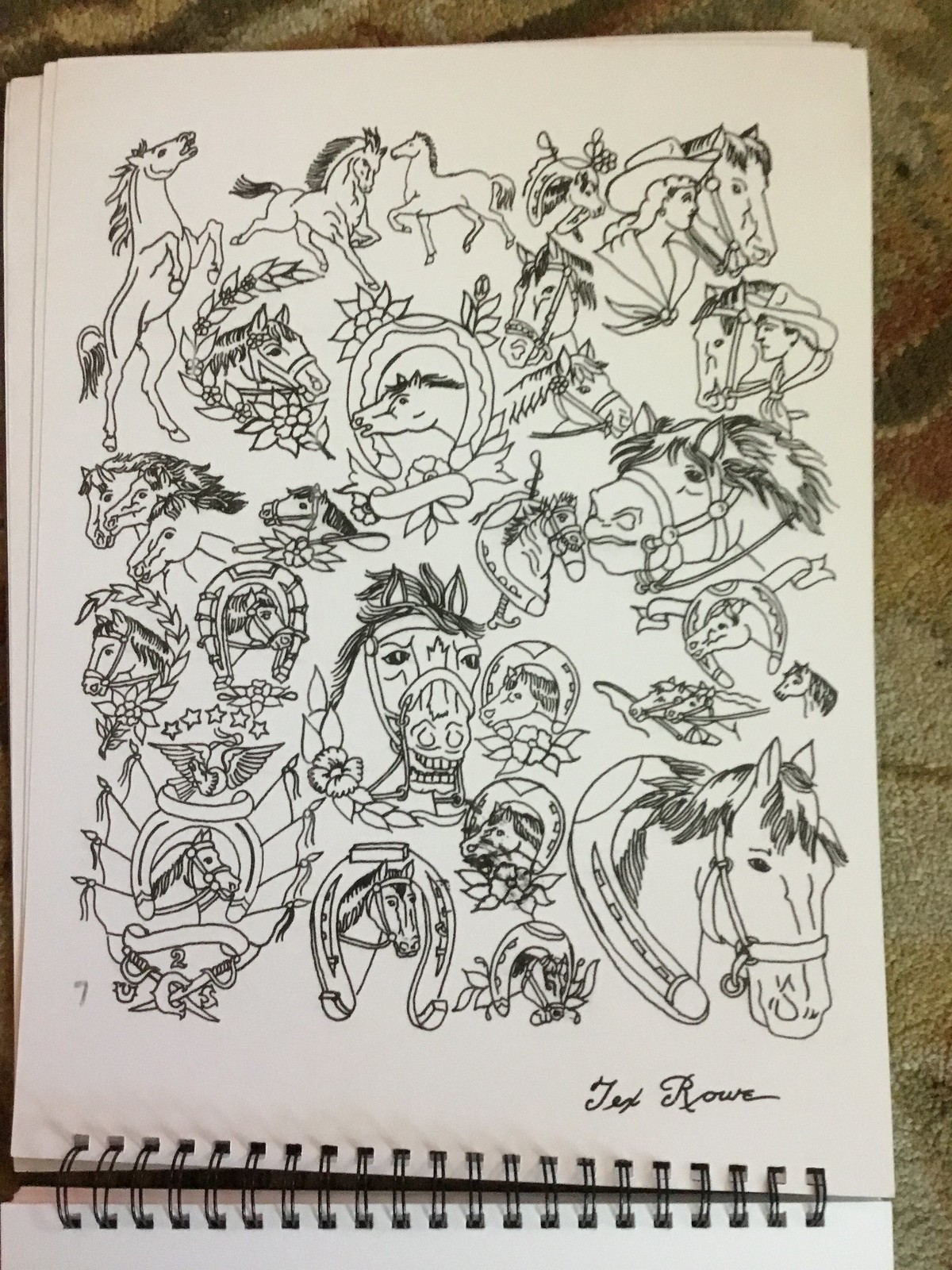The image depicts a page from a ring-bound, white sketchbook lying on a muted white-brown, patterned carpet. The page is filled with intricate black ink drawings of various horses and their heads. Prominently featured are multiple sketches of horse heads emerging from upside-down horseshoes, some adorned with flowers, and others positioned in wreaths. There is a horse rearing on its hind legs, a particularly aggressive-looking horse with its mouth open, and a framed horse with the number "2" below it. A detailed woman's portrait with a large hat and flowing hair, and a man with a hat and knotted scarf are situated in the upper left and right corners respectively, both next to horses. In the bottom right corner of the sketch, the artist's signature, "Jess Rowe," is visible.